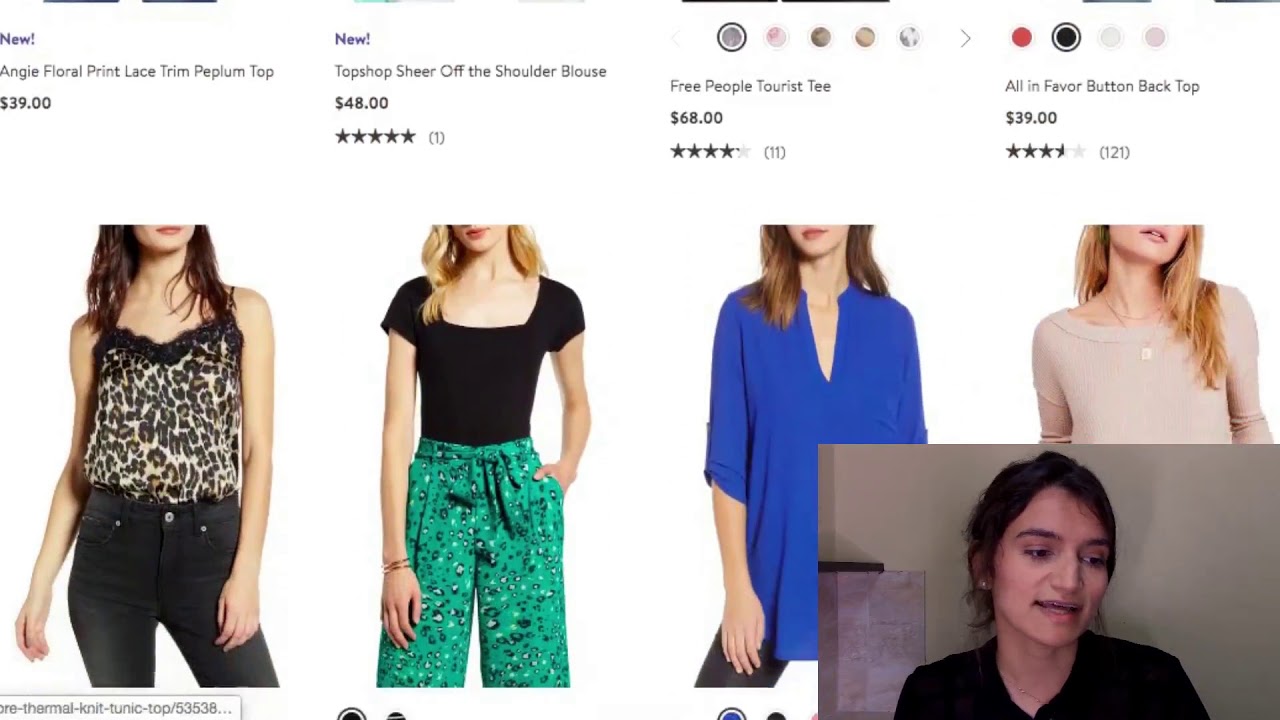The photograph depicts a person browsing an e-commerce website on their computer. The visible section of the webpage displays four clothing items, partially showing their images and labels. The items listed are:

1. "New! Angiofloral Print Lace Trim Peplum Top - $39."
2. "Off-the-Shoulder Blouse - $48," which has a five-star rating.
3. "Free Pupil Tierist Tee - $68," available in different color options. 
4. "Back Top - $39," shown in black and also offered in other colors.

Below these listings, there is a series of cropped photos featuring women modeling clothing. The images cut off the women’s faces just above the mouth, so only their outfits are visible. The first woman on the left is wearing an animal print top paired with black jeans. The second woman is dressed in a black top and bright green pants with a bow detail around the waist. The third woman is sporting a long blue top that extends to her thighs, while the fourth woman on the far right is in a scoop-neck cream or light tan shirt.

Additionally, there is a small video inset on the webpage showing a woman who appears to be live streaming. She has dark brown hair and is possibly of Middle Eastern or Indian descent. She is wearing a black v-neck top and is sitting against a white wall, seemingly focused on what’s displayed on the screen. It suggests that she may be providing a commentary or walkthrough of the e-commerce site.